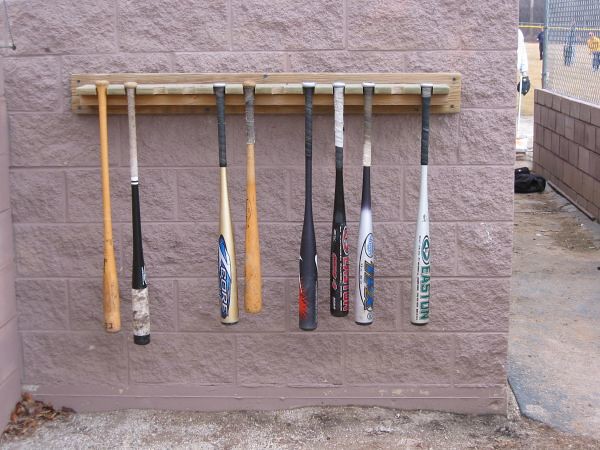This is a colored photograph capturing a scene at a baseball or softball field. Featured prominently in the foreground is a stone wall, which has a light pinkish-gray, tan-brown hue, or a light purple-brown color, adding to the rustic texture of the environment. Mounted on this wall is a wooden rack designed to hold baseball bats, securely nailed and meticulously holding eight distinct bats, each hanging upside down.

The bats vary in both material and design: some are metal while others are wooden. Specific details include a brown bat, a black bat with a white handle, a bat with a striking black and gold design with blue on the end, another simple brown bat, a black and red bat, both a black and red bat, and one with a black handle and a white body featuring green on the end. Their varying lengths and vibrant colors add visual interest to the image.

Below the rack, the concrete walkway is visible, and the presence of leaves towards the corner of the paddock suggests the season might be fall, complemented by patches of sand and dirt. In the background to the right, past a chain-link fence and a shorter wall, players, possibly children, are seen indicating a casual game or practice session, providing a lively context to the image. This scene beautifully captures the essence of a community baseball field, steeped in activity and seasonal subtleties.